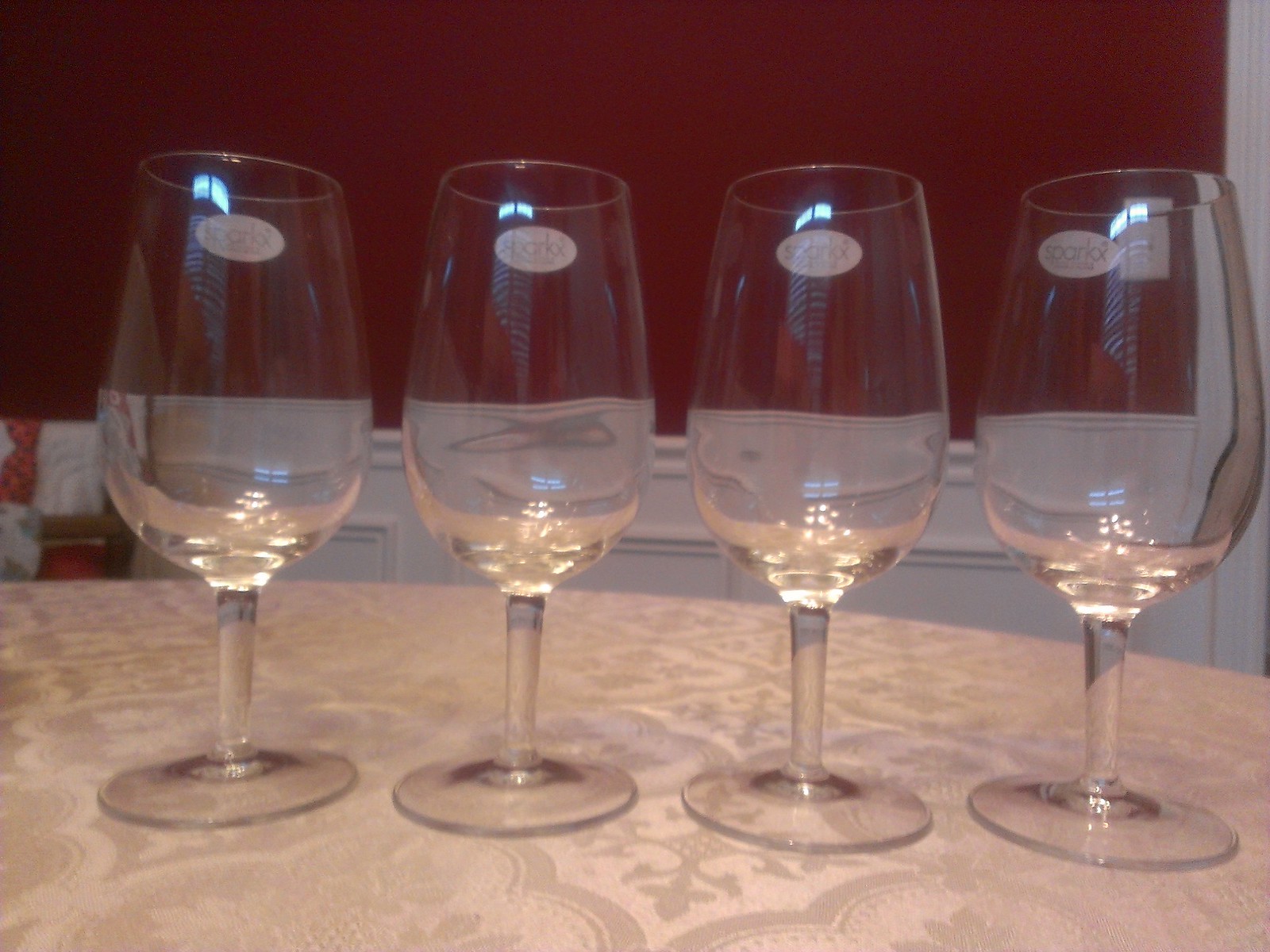The photograph captures four empty wine glasses, each with medium-sized stems and tall, clear glass bowls, arranged in a neat row on a table adorned with a cream-colored tablecloth. The tablecloth features an intricate square design interspersed with floral motifs, embossed in a slightly darker shade of cream. The glasses are of identical style and size, each bearing a logo, though it is unclear whether the logos are etched on the glasses or merely a part of a reflection from the environment.

The background features a distinctive two-tone wall, with a dark maroon section extending down from the ceiling and transitioning into a lighter grey hue below. To the left, there is an object with an alternating pattern of red and grey, possibly a decorative piece or a furniture item. On the right side, a grey structure ascends to the ceiling, potentially a door, but it is not fully visible within the frame. The lighting in the scene casts minor reflections and possible light tricks, giving an impression of stains on the tablecloth behind the glasses. This careful arrangement and detailed setting suggest a restaurant ambiance, creating a refined and serene atmosphere.